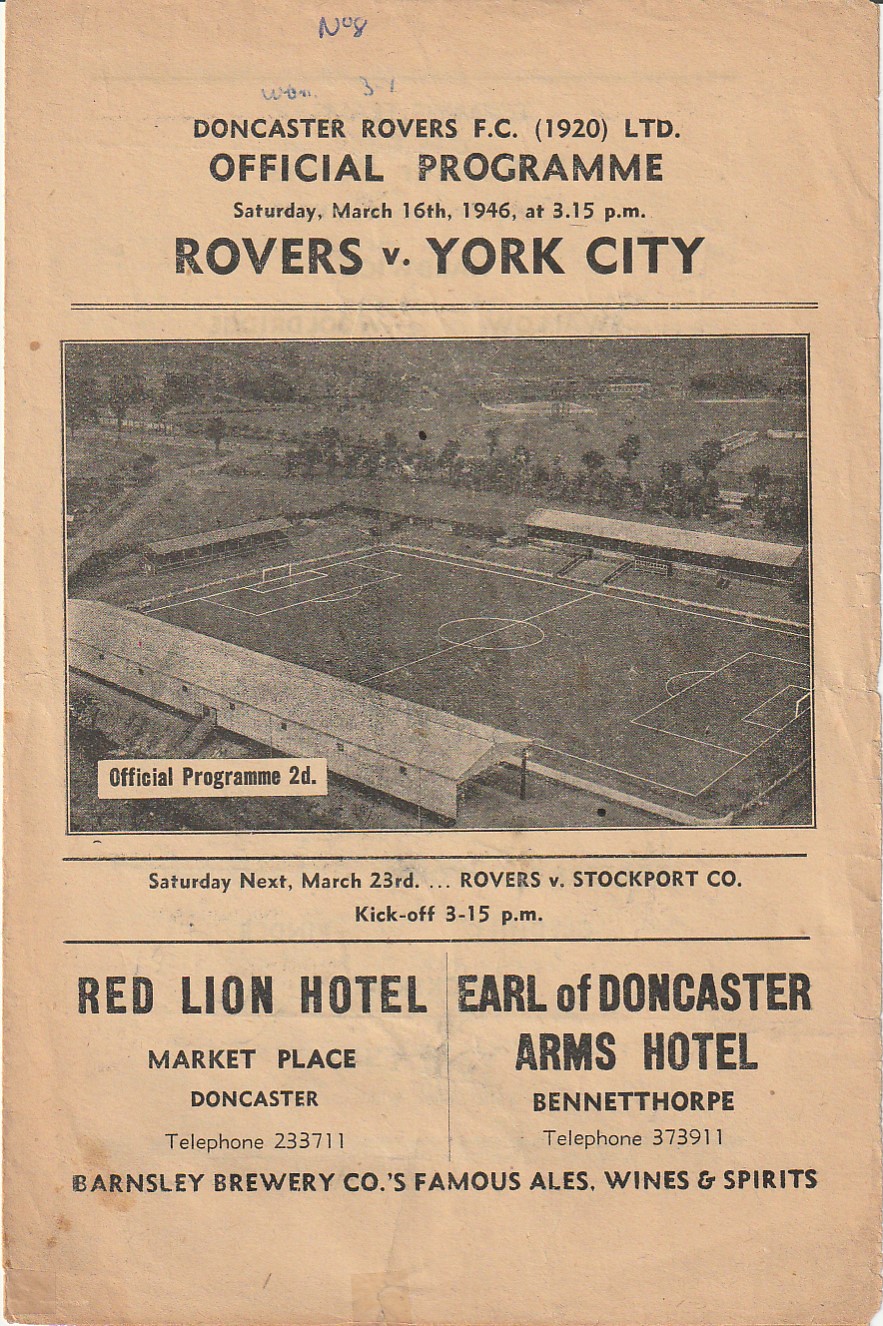This image features an old and weathered program for a Doncaster Rovers FC football match, with a somewhat yellowed top and black font. The program, dated Saturday, March 16, 1946, at 3:15 p.m., announces a match between Doncaster Rovers and York City. Below this text is an aerial black-and-white photograph of a soccer field, labeled "Official Program 2d" in the bottom left corner. The image depicts the stadium, surrounding greenery, and local landmarks. Underneath the photo, another match is advertised for the following Saturday, March 23, 1946, where Rovers will play against Stockport Co. at 3:15 p.m. 

In the lower section of the program, there are two divided ads: the left one promoting Red Lion Hotel, Marketplace, Doncaster (telephone 233711), and the right one for Earl of Doncaster Arms Hotel, Bennetthorpe (telephone 373911). At the very bottom, in larger text, an ad for Barnsley Brewery Company's famous ales, wines, and spirits is prominently displayed. Throughout, the text is presented in various black fonts and styles, contributing to the program's vintage appeal.